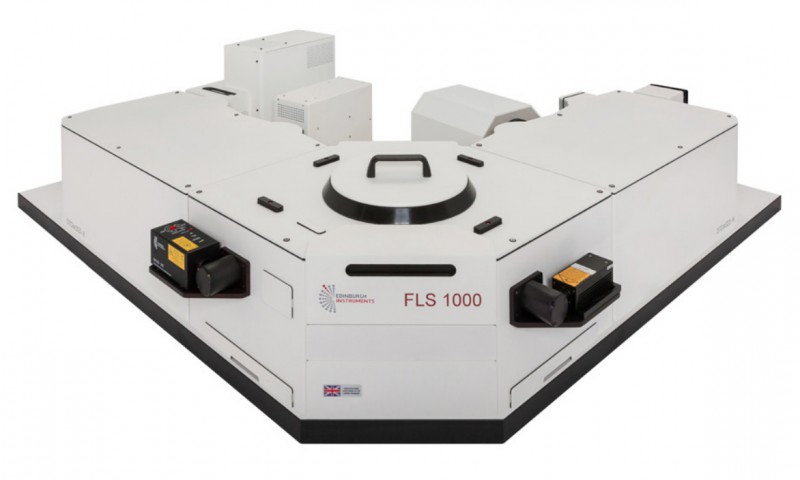The image shows a piece of machinery or possible medical equipment set against a white background, labeled with "Edinburgh Instruments" and "FLS 1000" in red lettering. This apparatus, primarily light beige with a black base, is L-shaped and features a top circular component with a black handle. Black rectangles and cylinders protrude from both sides. Though out of focus, additional components seem to be at the back, resembling computer parts or motors, and one side bears elements that appear to be yellow. The machine has no discernible scale and includes a British flag logo at the bottom front.